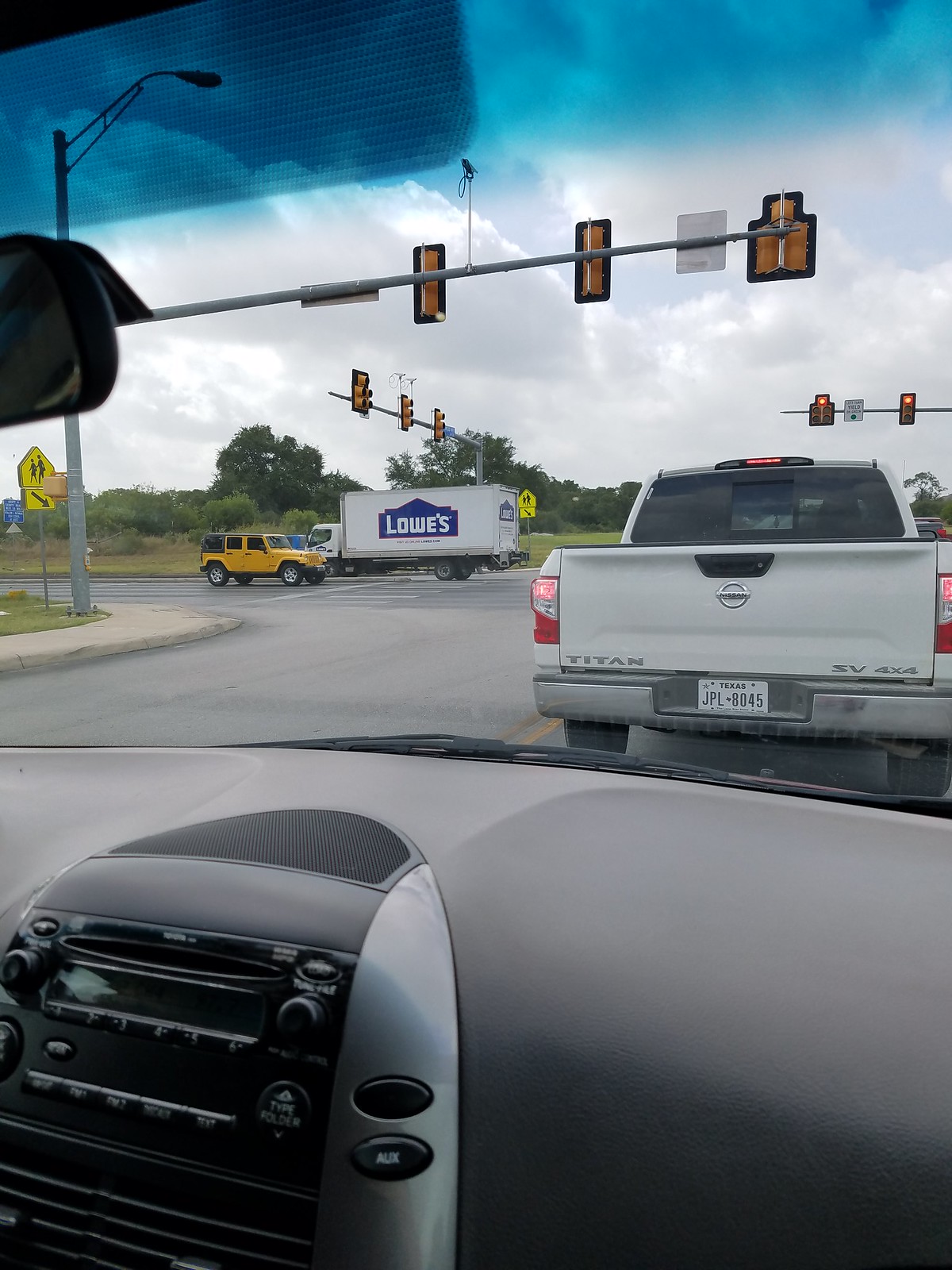This color portrait photograph captures the viewpoint from a passenger inside a vehicle at an intersection on an overcast day. The vehicle’s dark to light gray dashboard spans the bottom of the image, featuring the infotainment system with a visible AUX button and a speaker grill. A single black windshield wiper rests at the base of the windshield. Beyond the windshield, the street scene unfolds with a silver pickup truck directly ahead, a white and blue Lowe's truck moving perpendicular to the left, and a yellow Jeep also to the left. Iconic horizontal scaffolding-type poles support yellow-framed traffic signals, with the backside of one such signal prominently in view. The left side reveals a red traffic light, a sidewalk, and some greenery with grass and trees. Above, the sky is filled with a mix of white and gray clouds, hinting at the overcast weather.